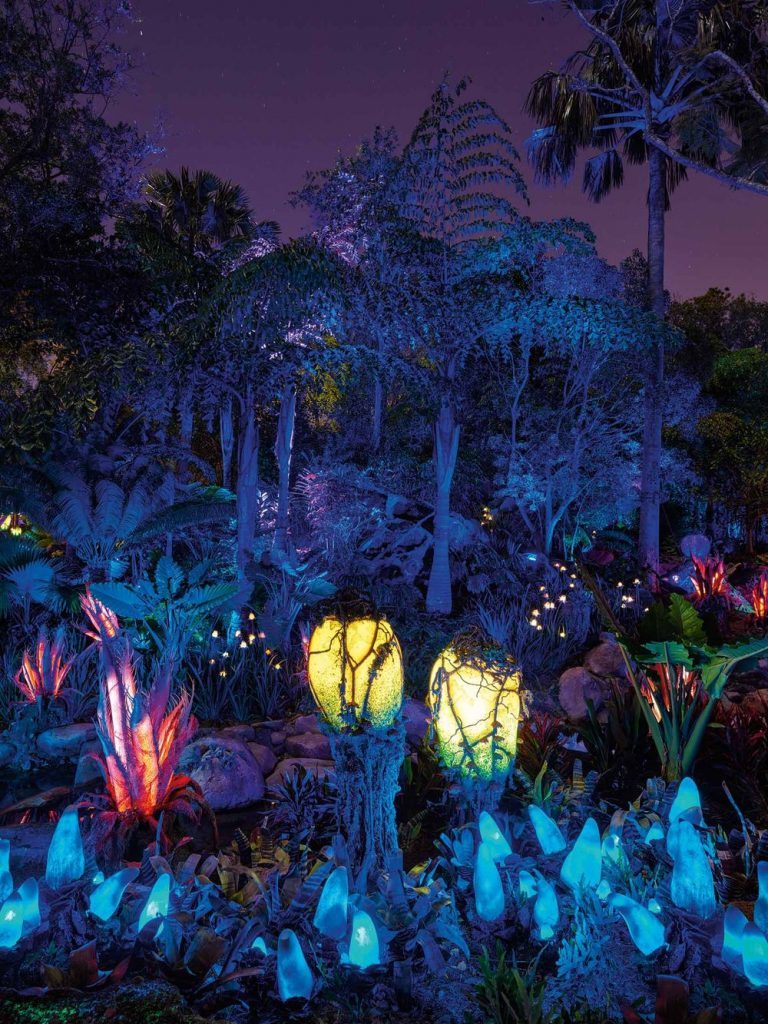The image depicts a serene nighttime garden scene illuminated by an array of colorful lights. The sky overhead is a striking purple, likely due to overcast conditions. The garden is adorned with various types of plants, including green trees and a palm tree. Blue lights prominently feature at ground level, casting a serene glow in the foreground. In the background, there are red and yellow lights, as well as two striking yellow floodlights illuminating ornamental features. Pink lights can also be seen on the left side, adding to the colorful tapestry. The scene exudes a peaceful ambiance, reminiscent of an amusement park or a nature garden, with no animals or people present to distract from the vibrant, artificial yet tranquil illumination.